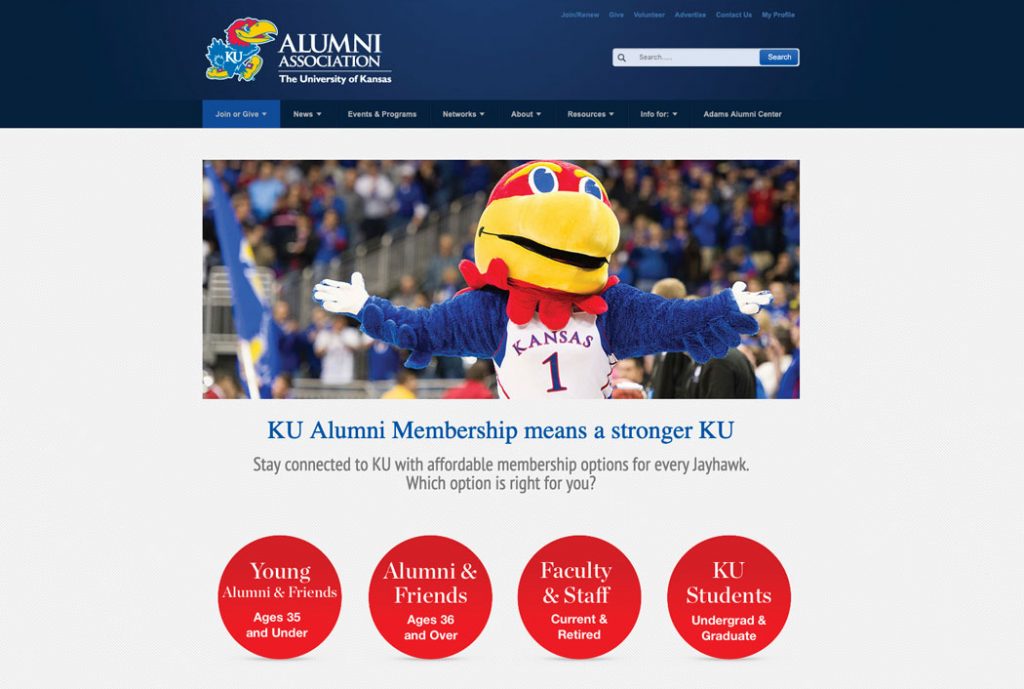The image features a dark blue header with a depiction of the iconic Jayhawk mascot—a woodpecker with a striking red head, a bright yellow beak, and a blue chest emblazoned with the letters "KU". Beneath this logo, bold white capital letters read, "Alumni Association," accompanied by "University of Kansas" below it. Adjacent to these texts on the right is a search bar. Spanning the header is a menu bar with eight dropdown options, although the specifics are too small to discern.

Directly below the header, the main content area showcases a vibrant image of the Jayhawk mascot live on the basketball court amid an electrifying game. The mascot sports a white jersey with "Kansas" and the number "1" proudly displayed on the front. The background reveals packed bleachers filled with an enthusiastic crowd.

Below the image, in prominent blue text, the statement "KU Alumni Membership means a stronger KU" is presented. This is followed by gray text offering details: "Stay connected to KU with affordable membership options for every Jayhawk. Which option is right for you?" Underneath this text, four circles contain white text with the following categories: "Young Alumni and Friends ages 35 and under," and "Alumni and Friends ages 36 and under."